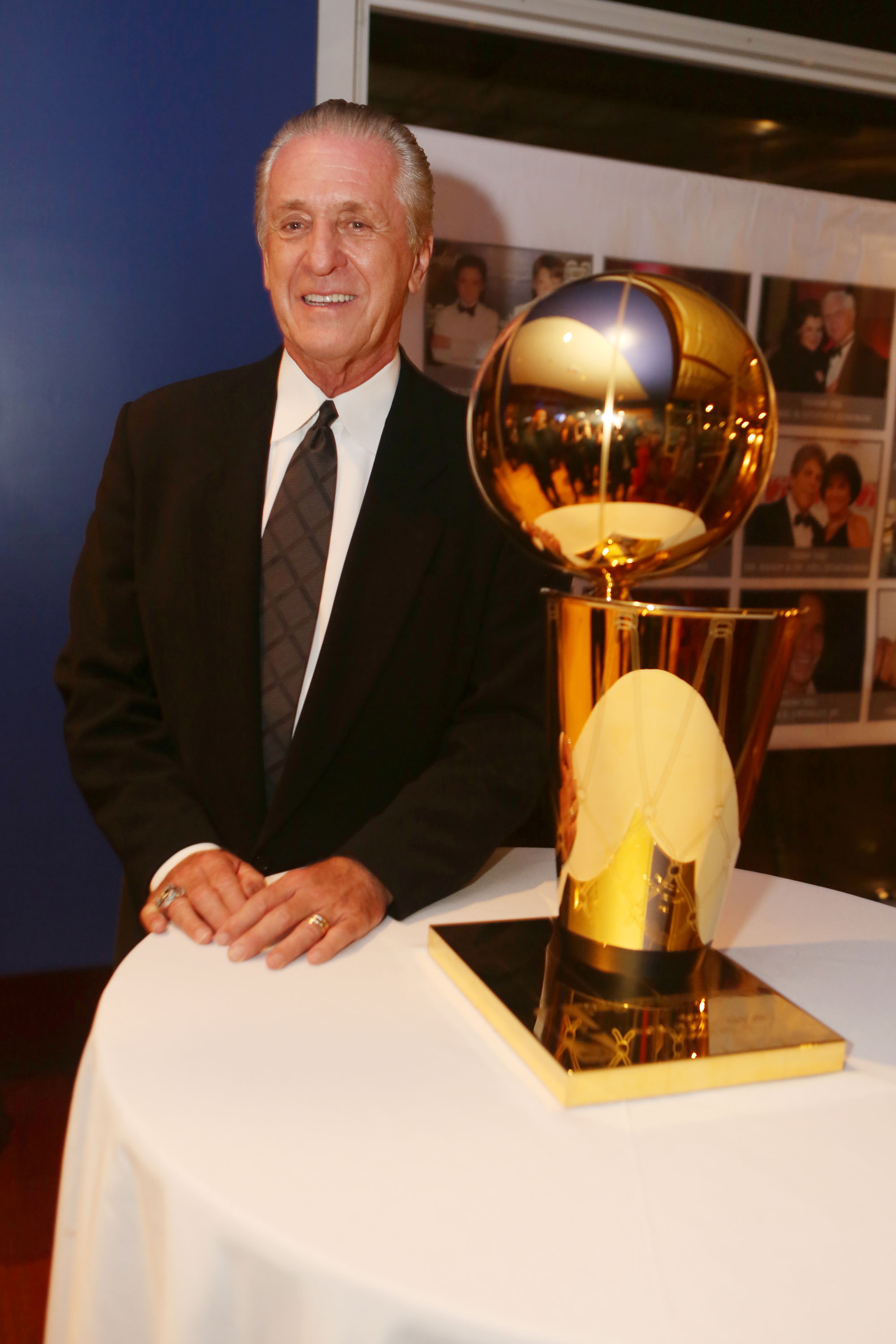In the image, an older, distinguished gentleman, likely a famous actor, is seated contentedly at a round table covered with a pristine white tablecloth. He is all smiles, his short, white hair slicked back neatly. He dons a sophisticated black suit paired with a crisp white button-up shirt and a distinctive brown tie adorned with a diamond pattern. Silver rings gleam on his ring fingers as he rests his arms on the table, drawing attention to the golden trophy that stands majestically at the table's center. The trophy, with its shining golden base and intricate design, features a narrow cup-like structure with a reflective, universe-themed top. The mirror-like top catches the light and provides a fragmented reflection of several people and couples in the background, hinting at a larger celebratory event.